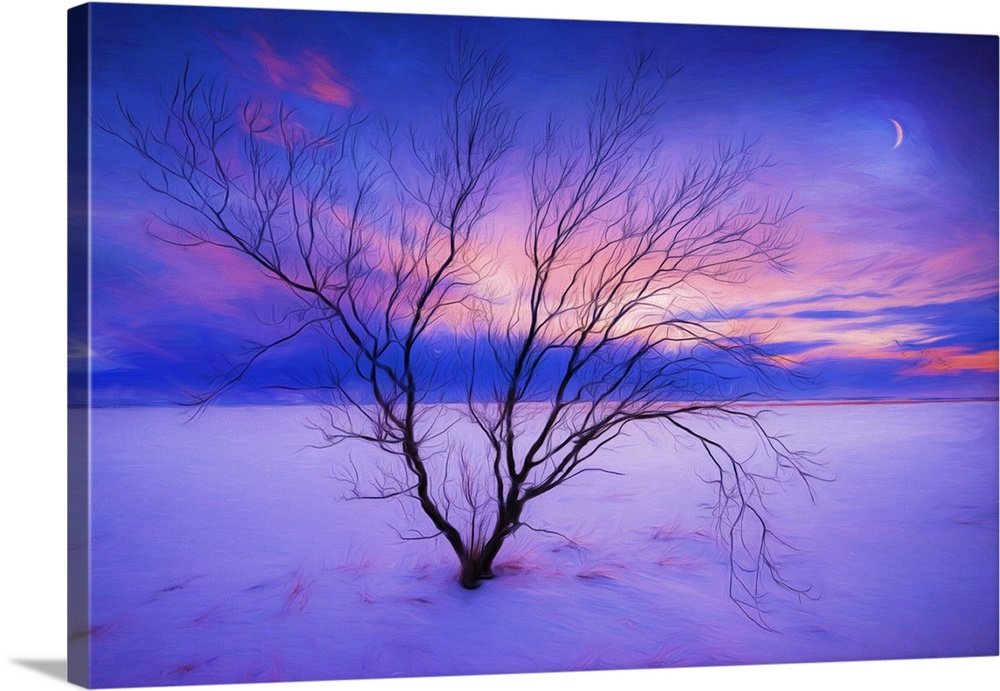The photograph captures a poignant canvas painting displayed upright against a flush white background. The canvas casts a subtle shadow to the right, hinting at a light source from that direction. The painting itself is of a beautifully haunting winter scene: a withered tree, bare of leaves, standing solitary in the foreground of a vast, snow-covered field. The snow stretches into the distance, where it meets a striking skyline. The sky transitions from dark blue and lavender to shades of orange and yellow, suggesting a sun that has just set behind distant clouds, while a crescent moon occupies the upper right corner. Wisps of clouds add texture to the serene twilight sky. Though carefully crafted, the painting bears no signature, evoking a sense of anonymous artistry. Thin patches of grass struggle through the snow near the tree, adding subtle detail and depth to the wintry landscape.